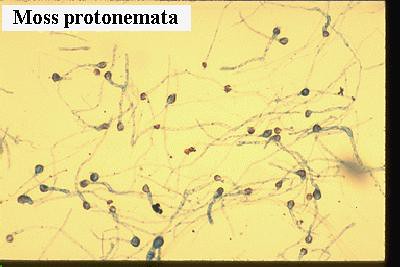This image appears to be a printout of something observed under a microscope, characterized by a tan or yellowish background. The border of the image is black, with the right side being noticeably thicker than the bottom. In the top left corner, a small white rectangle contains the black text "MOSS PROTONEMATA" (M-O-S-S P-R-O-T-O-N-E-M-A-T-A). The primary focus of the image is a collection of microscopic structures resembling sperm cells or spores, displaying black heads and semi-transparent, elongated tails. These structures, referred to as moss protonemata, are dispersed randomly across the image, creating a chaotic array of dark, tadpole-like figures.